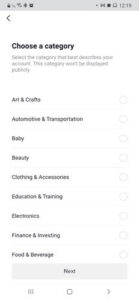This image is a low-quality, blurry screenshot taken from a mobile phone. The top section of the screenshot displays a gray notification bar containing various icons, although they are too blurry to distinguish clearly, except for the visible time which reads 12:18. Below this notification bar, the screen transitions to a predominantly white interface.

In the upper-left corner of this white screen, there is a small left-pointing arrow icon. Directly beneath the arrow, a bold black text heading reads "Choose a category." A gray, barely legible sentence follows this heading, likely starting with the word "Select."

The main portion of the screen features a list of categories in black font, clearly readable, arranged as follows:

1. Arts and Crafts
2. Automotive and Transportation
3. Baby
4. Beauty
5. Clothing and Accessories
6. Education and Training
7. Electronics
8. Finance and Investing
9. Food and Beverages

These categories are listed in a straightforward column, intended to guide the user to different sections of the application or website related to various interests and needs.